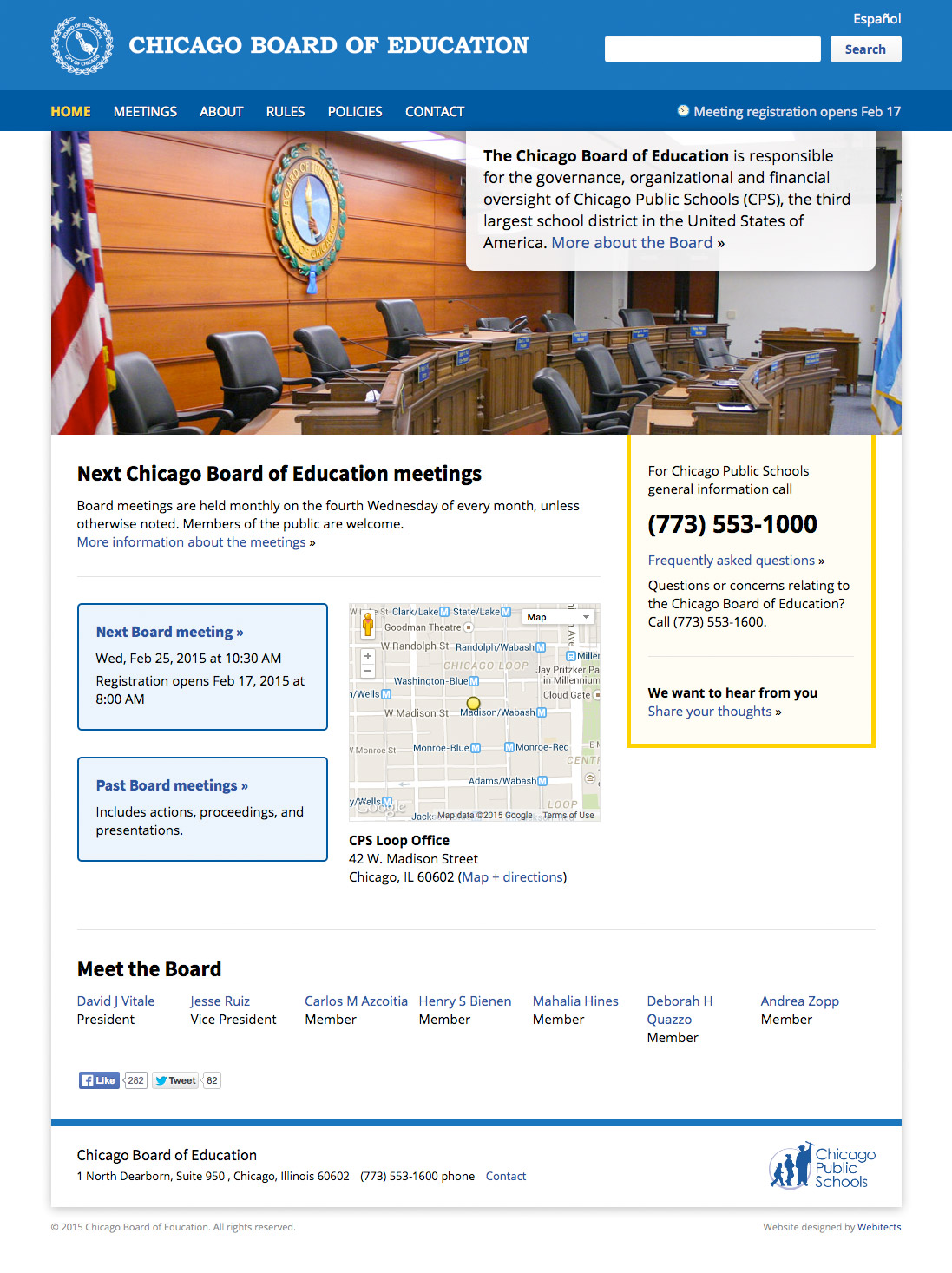The image features a webpage dedicated to the Chicago Board of Education. On the right side, there is a prominently displayed search bar. At the bottom, a menu includes sections such as Home, Meetings, Rules, Policy, and Content. Beneath this menu, there is a picture of an empty room, which appears to be a meeting or conference space. In the backdrop, an American flag is visible, symbolizing governance and patriotism. 

The webpage announces upcoming Chicago Board of Education meetings, featuring two small boxes that specify the dates and times of these events. There is also a button for accessing details of past board meetings. To the left of this section is a map pinpointing the location of the CPS Loop Office, along with the relevant meeting times. Below the map, there is information about where to find the general contact number. Finally, there is a section below this where visitors can ask questions and learn how to meet the board members.